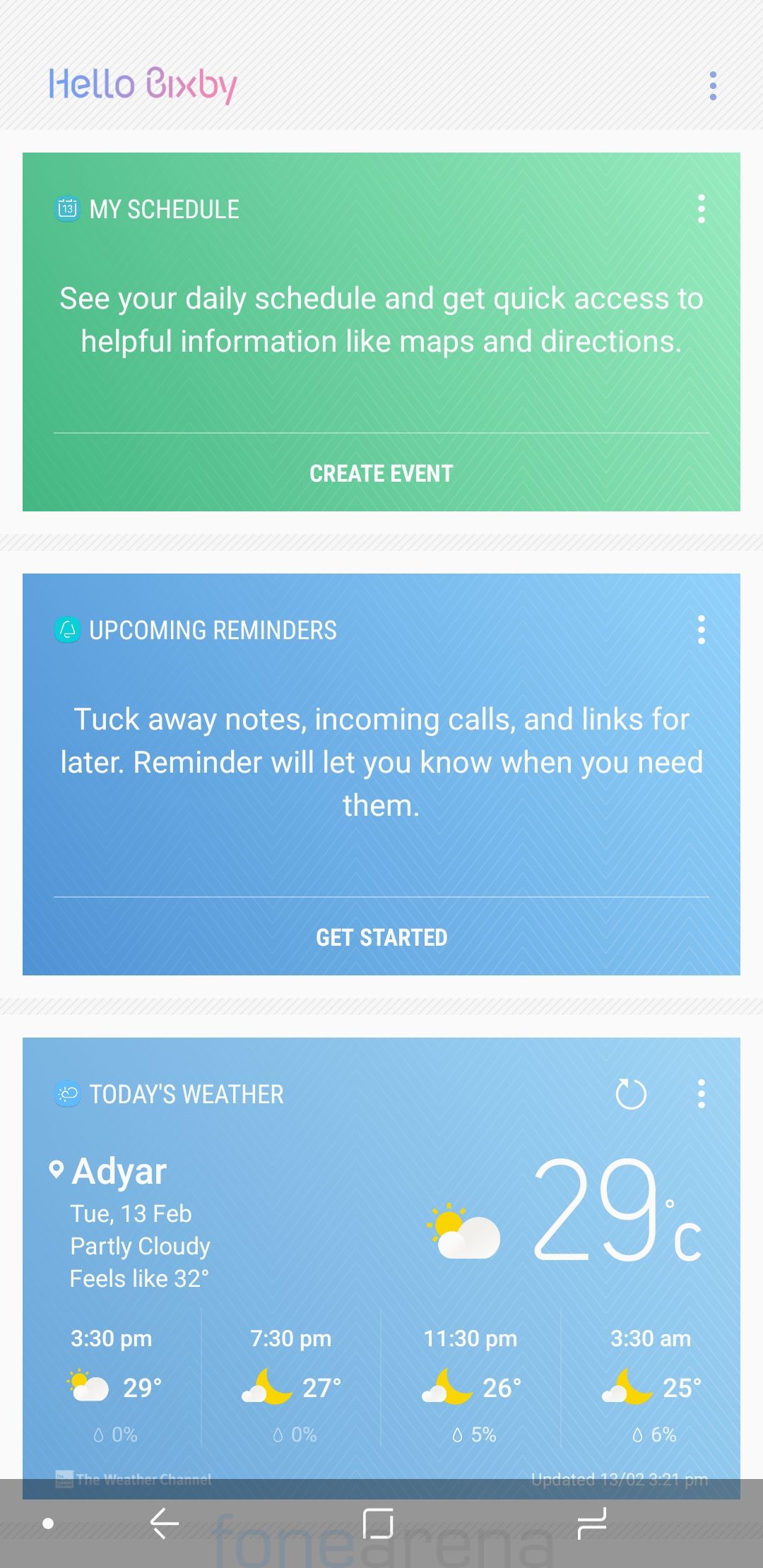The image showcases a vibrant Bixby app interface against a textured light gray background with subtle stripe patterns. At the top, the phrase "Hello, Bixby" is displayed in an ombre gradient, transitioning smoothly from light blue to purple and then to pink. Positioned to the right of this greeting is a three-dot icon, indicating a dropdown menu.

Below, there is a rectangular section with an ombre hue, transitioning from dark green in the bottom right to light green in the upper left. This section features white, capitalized text stating "MY SCHEDULE," accompanied by a blue calendar icon on the left. Directly below, it reads, "See your daily schedule and get quick access to helpful information like maps and directions." This section is also equipped with a three-dot dropdown menu icon located at the top right. A thin, light border encases this area, followed by the bold text "CREATE EVENT."

Further down, there's another large rectangular area. This section features a very subtle ombre transition from light blue to dark blue, almost indiscernible. It contains white, capitalized text displaying "UPCOMING REMINDERS." To the left, there's a bell icon on an aqua background, suggesting notifications. Within this section, it details: "Tuck away notes, incoming calls, and links for later. Reminder will let you know when you need them." Below this, another faint divider precedes the bold text "GET STARTED," written in capitalized white lettering.